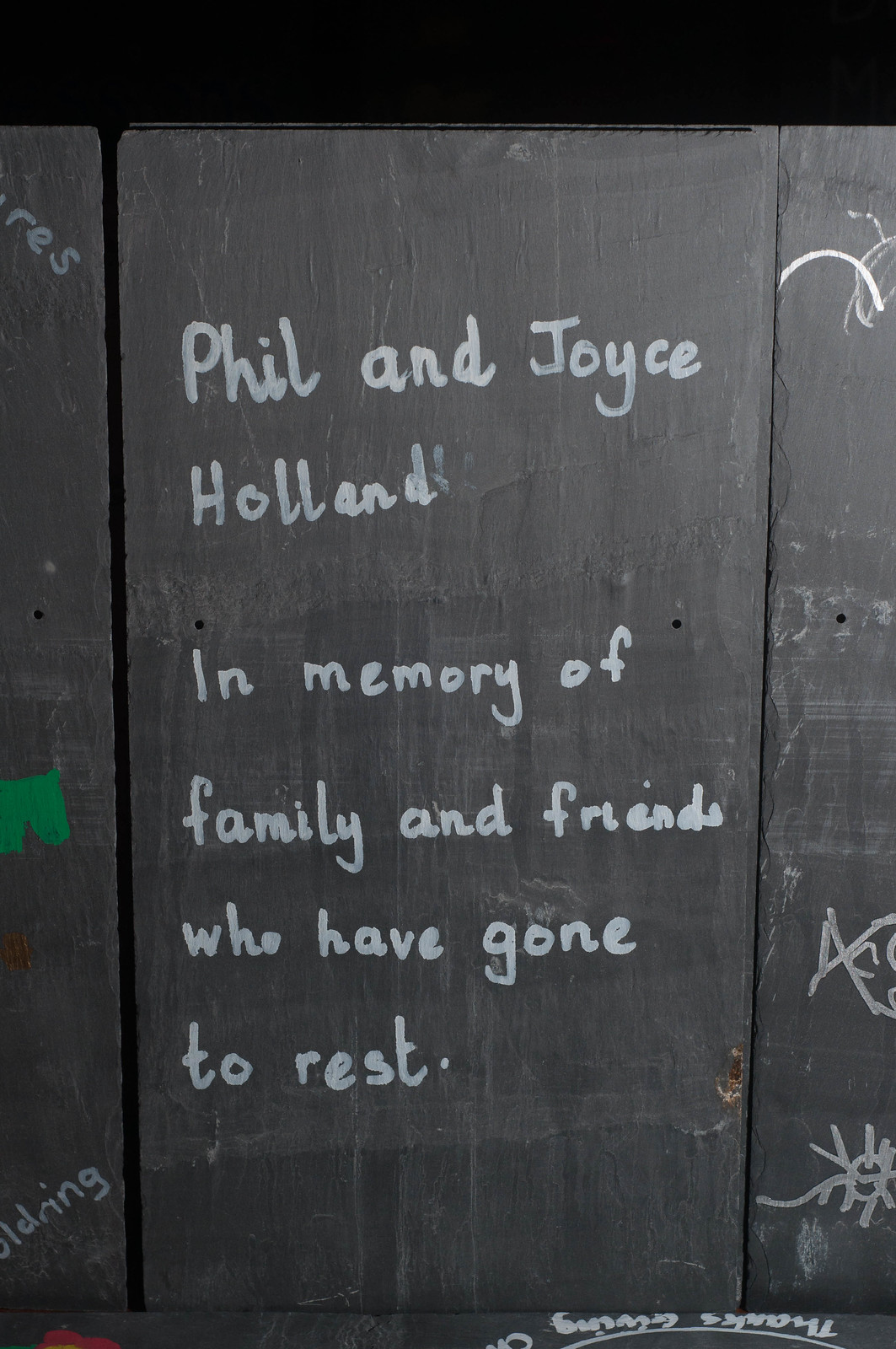The image showcases a series of vertically aligned, gray-black painted boards, resembling a fence. The central board dominates the scene, extending from top to bottom. Prominently, in white lettering at the top, it reads, "Phil and Joyce," followed by "Holland" on the next line. Below, there is a space before the inscription continues with, "In Memory of," then "Family and Friends," followed by "Who Have Gone," and "To Rest." To the right of the central board, partially visible white markings suggest additional symbols and writing, though they are too faint and small to decipher clearly. On the left side of the central board, there is a distinct green painted image, resembling a pair of shorts or possibly a horse head, along with the partial lowercase letters "RES" at the top and "L-D-N-I-N-G" at the bottom. Additional white writing appears at the very bottom right of the picture but is too blurred to make out, potentially being a name in cursive.